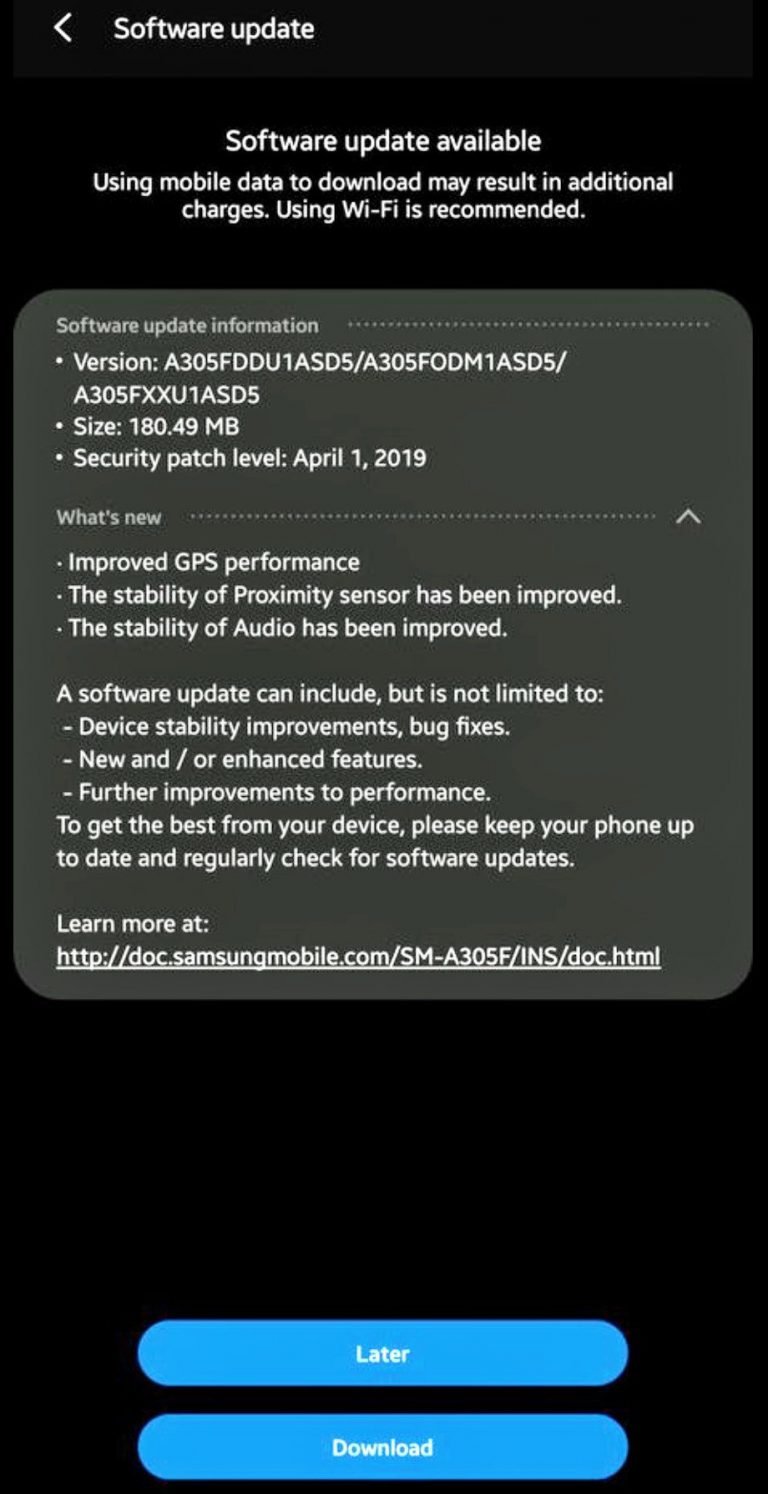The image depicts a black rectangular notification detailing a software update, likely on a mobile phone. At the top of the rectangle, there is a left-facing arrow next to white text reading "Software Update." Below this, there is a noticeable triple space followed by the text "Software Update Available" in white. The subsequent lines state: "Using mobile data to download may result in additional charges. Using Wi-Fi is recommended," with each sentence centered within the black rectangle.

Further down, after a double space, there is a light gray square featuring the text "Software Update Information." Beneath this heading are four lines followed by the gray text "What's New," which introduces seven listed items in white. Finally, there is a double space before a URL for more Samsung information, which is underlined.

At the bottom of the rectangle, there are two blue buttons with white text: the left button reads "Later," and the right button reads "Download."